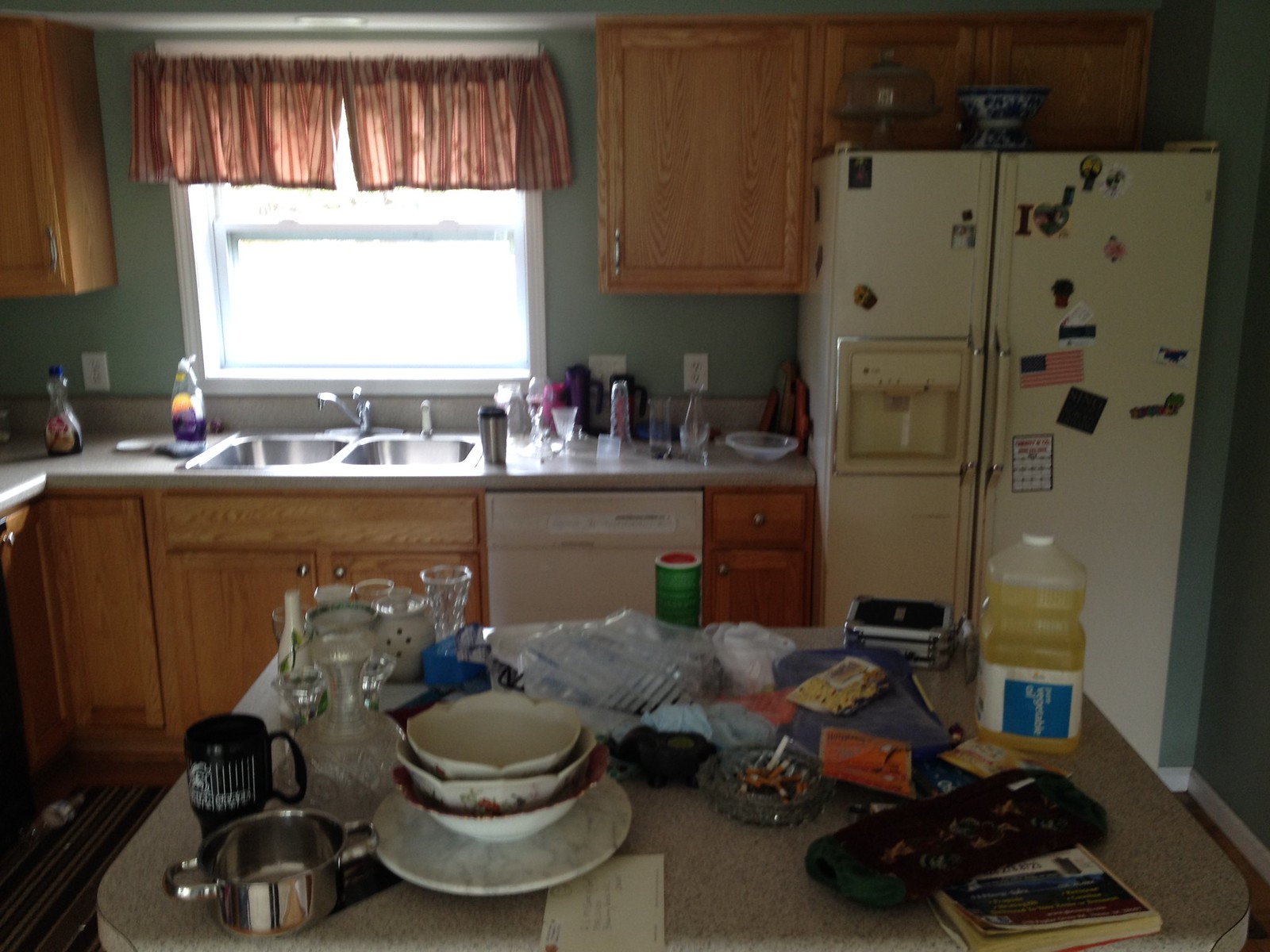This photograph captures a vintage 1980s-style kitchen, characterized by its warm, honey-blonde wood cabinets that feature sleek silver handles. The kitchen layout includes an L-shaped counter prominently situated in the middle and extending to the back of the room. To the right, a refrigerator is seamlessly integrated into the cabinetry, which extends above and to the left of the appliance, as well as to the right of a double basin sink. The sink is equipped with a separate sprayer and is positioned beneath a window adorned with a vertically striped valance in shades of pinkish-orange and beige.

On the L-shaped counter to the left of the sink, a purple bottle of liquid dish soap is noticeable. Various scattered dishes, cups, and a few cutting boards leaning against the refrigerator populate the counter space to the right of the sink. A silver travel mug sits on this side as well. Adjacent to the sink, an ivory-colored dishwasher adds to the vintage aesthetic.

In closer view, a table at the forefront of the image draws attention. This table, an old laminate piece echoing the 1980s vibe, holds an eclectic mix of items. There is a bottle containing a yellow liquid, a squared-off jug, and a green cardboard canister of grated parmesan cheese. An ashtray, filled with several cigarettes, rests nearby. A stack of bowls atop a small plate, a very small saucepan with two round handles, and another black plastic travel mug are casually arranged. Also present is a sophisticated-looking crystal vase, accompanied by several other crystal and ceramic items occupying the back left corner of the table. Completing the scene is a book resembling a notepad and an envelope featuring an address label, rounding out the domestic tableau with a touch of everyday life.